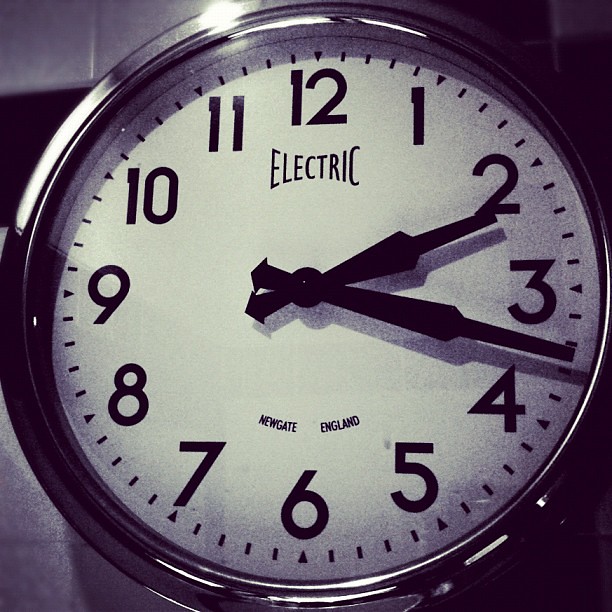This detailed photograph captures a square image with a prominently featured large vintage-style wall clock at its center, framed by what appears to be a stainless steel or silver rim. The background reveals a hint of a white brick wall, but the image is zoomed in enough that the clock dominates the view, and the right side of the photograph fades into black. The clock face is white, adorned with large black printed numbers and dash marks in between for precise time-telling. At the top, just below the number 12, the word "electric" is clearly visible, while at the bottom, just above the number 6, it reads "Newgate, England," suggesting an English origin. The hour and minute hands are designed like arrows, with broad bases that taper to thinner tips reminiscent of old-time cigarette holders. The hands are positioned to indicate a time of approximately 2:17.